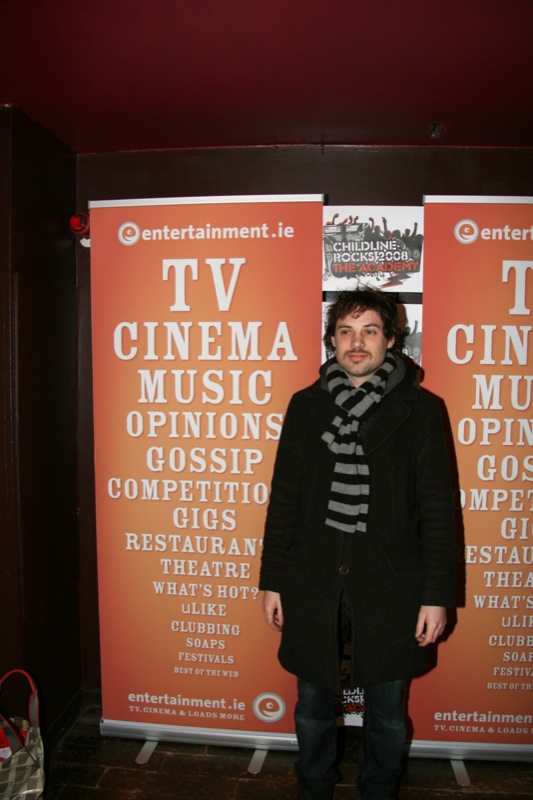This photograph captures a man posing at what appears to be an event, likely held at the lobby of a theater. The man occupies the lower left quadrant of the image, dressed in a black overcoat with a gray and black striped scarf draped around his neck. He has shaggy brown hair, a five o'clock shadow of a beard and mustache, and is wearing dark denim and possibly high boots. He’s gazing slightly to the side with a neutral expression.

Directly behind him are two identical backdrops with an orange background covered in white text, promoting the website entertainment.ie. The backdrop lines both sides of the man and features terms like "TV, cinema, music, opinions, gossip, competition, gigs, restaurant, theater, what's hot, you like clubbing, soaps, festivals, best of the web," prominently visible. The text overlays a combination of black and white, and orange imagery, including figures with raised arms. Additionally, the center part of the backdrop mentions "Child Line Rocks 2008 The Academy." The scene's background is predominantly black, highlighting the bright promotional displays behind the man.